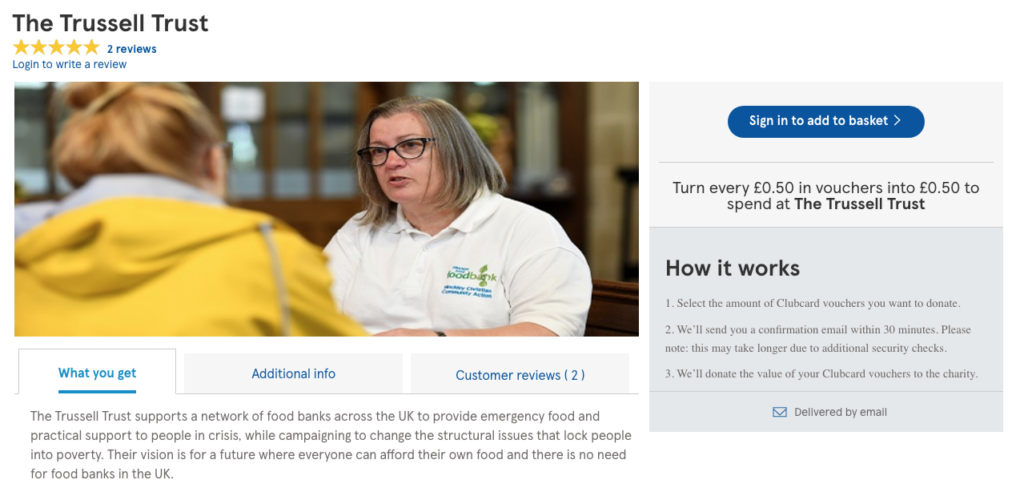The top section features a black header with the text "Trust Suit Trust" written in a sophisticated font. Adjacent to this text, there are five gold stars indicating a rating system. To the right of the stars, in blue text, it reads "2 reviews", and further to the right, a prompt in blue says "log in to write a review."

Below this, there is a rectangular section displaying two people engaged in a conversation. One person is shown from the back, revealing their dirty blonde or light brown hair styled in a bun. This individual is wearing a yellow long-sleeve jacket with a gray top underneath, and glasses. She is interacting with another person, visible from the front, who is wearing a white shirt labeled "Food Bank" and also has black glasses. The background of this section is gray, emphasizing the oval-shaped blue element in the foreground which reads "sign in to add basket" in white text. Beneath this, a gray line introduces the next section.

Following the line, black text describes a rewards system: "Turn every €0.50 in vouchers to €0.50 to spend at the Trust Suit Trust”. As the background shade deepens, an instructional guide titled "How it works" appears in black font. It details the process in three steps:
1. "Select the number of club card vouchers you want to donate to. We'll send you a confirmation email within 30 minutes. Please note this may take longer due to additional security checks."
2. "You will donate the value of your club card vouchers to charity.”

A blue envelope icon and the text "delivered by mail" are centered beneath another gray dividing line. On the left side, three tabs are displayed: the first tab highlights "What you get" in a blue underline against a white background. The next two tabs, labeled "Additional info" and "Customer reviews and privacy," are in blue text on a gray background. 

This detailed layout provides a comprehensive look at the trust and review system, visual composition, and functional instructions for utilizing vouchers and donations.